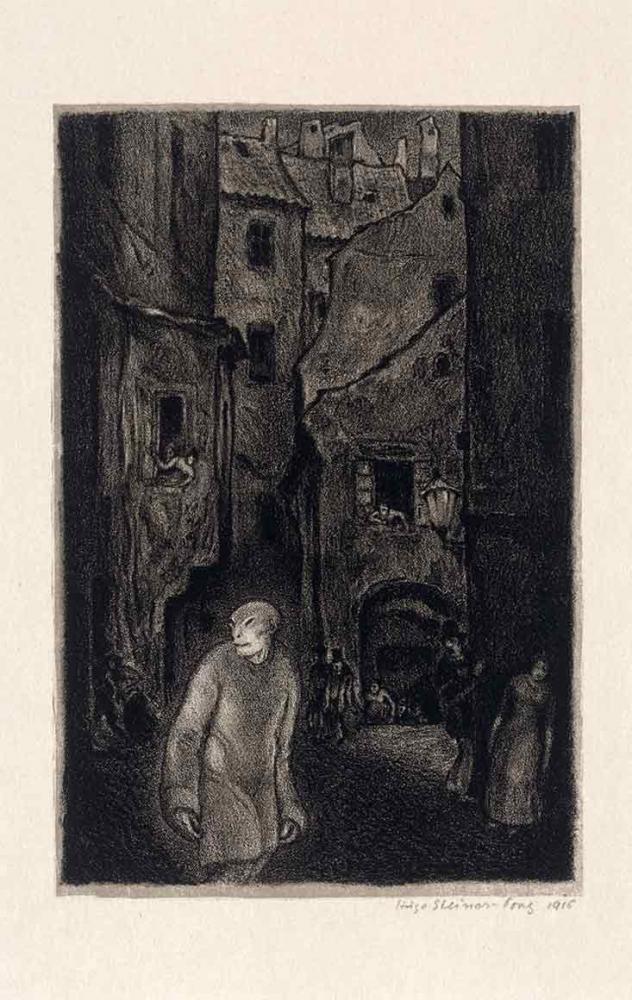This detailed black and white artwork, possibly created with charcoal or pencil, portrays a surreal cityscape from 1915, as indicated by the artist's signature and date at the bottom. It features an eerie humanoid figure with elongated, oval eyes and alien-like facial features, dressed in a long coat, positioned prominently in the foreground. The background reveals an old, curvy, and somewhat dilapidated city with tall buildings. The buildings have numerous windows from which curious people gaze at the peculiar figure. On the streets below, other individuals also react in astonishment or apprehension, with one person notably trying to hide behind the corner of a building. The image is set against a tannish background, enhancing its dark and intricate details.